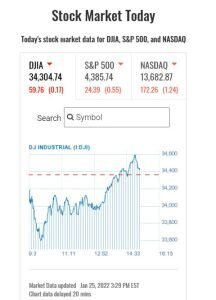**Websites Section - Detailed Stock Market Data Display**

In this extremely tiny and hard-to-read image, the heading reads "Stock Market Today," followed by a sub-heading that states, "Today's Stock Market Data for DJIA, S&P 500, and NASDAQ." Below this heading, the data is presented as follows:

- **DJIA**: 34,304.74, showing a decrease of 17%
- **S&P 500**: Down 0.5%
- **NASDAQ**: Down 1.24%

Below the market data, there is a search function where users can enter a stock symbol to perform a search. Underneath this section, a line graph is depicted, which oscillates frequently, reflecting the fluctuating market trends. The graph is annotated with the labels "Industries" and "Market Data." The entire snapshot is timestamped with the latest update on January 25th, 2022, at 3:29 p.m.